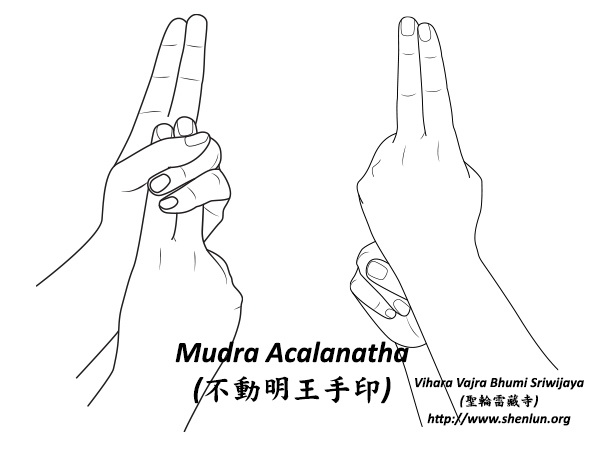The image features detailed, monochrome, computer-drawn line illustrations of two pairs of hands demonstrating specific sign language or symbolic hand gestures. Each pair of hands, positioned on opposite sides of the image, shows a left hand facing upwards with two fingers pointing straight up. Parallel to these fingers, the right hand threads its thumb through the ring and pinky fingers, with the remaining fingers extending upwards. In the center at the top, the text reads "Mudra Akalanatha," which appears to be a term related to these gestures and is challenging to pronounce. Below this central text, on the right side of the image, are the words "Vihara Vajra Bhumi Shri Vijaya," accompanied by additional text in Chinese or Japanese characters. At the bottom of the image, a URL, "http://www.shenyan.org," is stenciled in black and white, possibly linking to more information about the depicted gestures or the related cultural context.